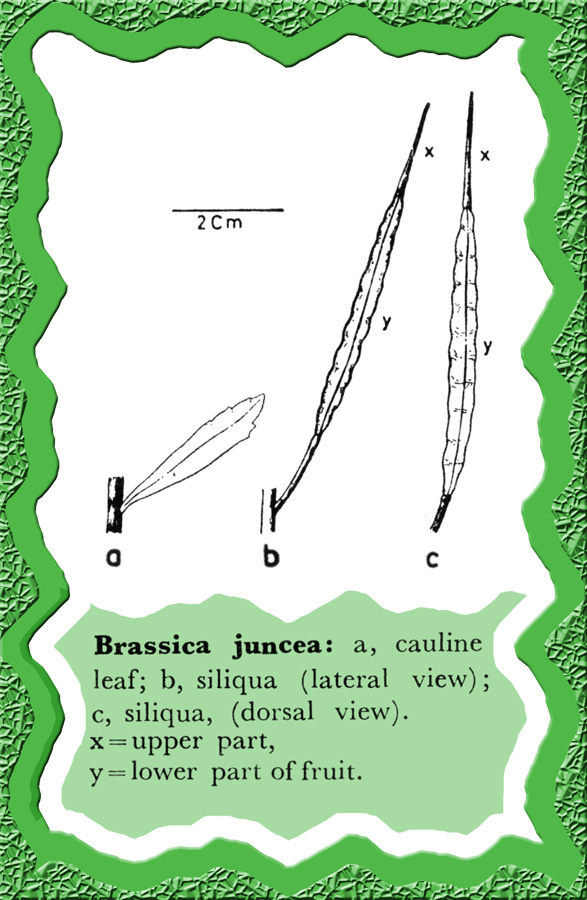The image depicts a detailed botanical diagram of the plant Brassica juncea, accompanied by explanatory labels. The large, rectangular graphic is bordered by an abstract, green, crocodile-skin-like texture with black outlines, resembling digitalized, raised paint. 

In the center, a white box showcases meticulous pencil or pen illustrations of the plant's parts. Three sections labeled A, B, and C depict different views: A features a small cauline leaf, B shows the siliqua in lateral view, and C presents the siliqua in dorsal view. The illustrations are framed by a rough-edged border, accentuating the central white space.

Within the white box, a scale marked "2 CM" provides reference, ensuring accurate interpretation of measurements. Letters X and Y are used to designate parts of the fruit, with X representing the upper part and Y indicating the lower part. Below these illustrations, in a green box with black text, the scientific notation reads: "Brassica juncea. A, cauline leaf; B, siliqua, lateral view; C, siliqua, dorsal view. X = upper part, Y = lower part of fruit."